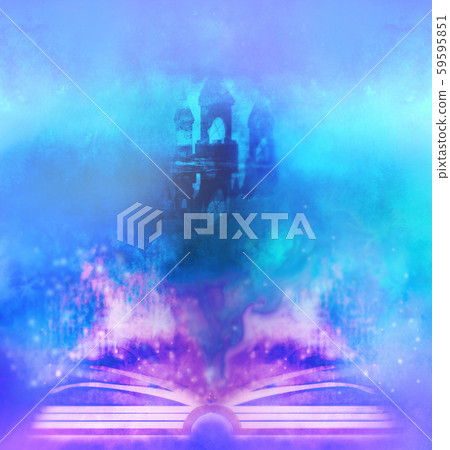In this surreal and dreamy image, a thick, open book with white pages and a pink cover lies prominently in the foreground. Several pages appear to be magically turning, some even lifted into the air, illustrating a mystical event. Ethereal, translucent flames in shades of pink and purple emanate from the book, accentuating its fantastical quality. The background features a foggy scene dominated by a faded, enigmatic castle with three pointed steeples, barely visible through the dense, blue-pink mist that engulfs it. The majority of the image is bathed in hues of blue and light green with subtle tints of pink and purple, creating a tie-dye effect. In the center, the text "P-I-X-T-A" in white is prominently displayed, accompanied by three hollow squares stacked diagonally, adding to the otherworldly atmosphere. The entire composition exudes an enchanting, fantasy-like aura that captivates the viewer's imagination.